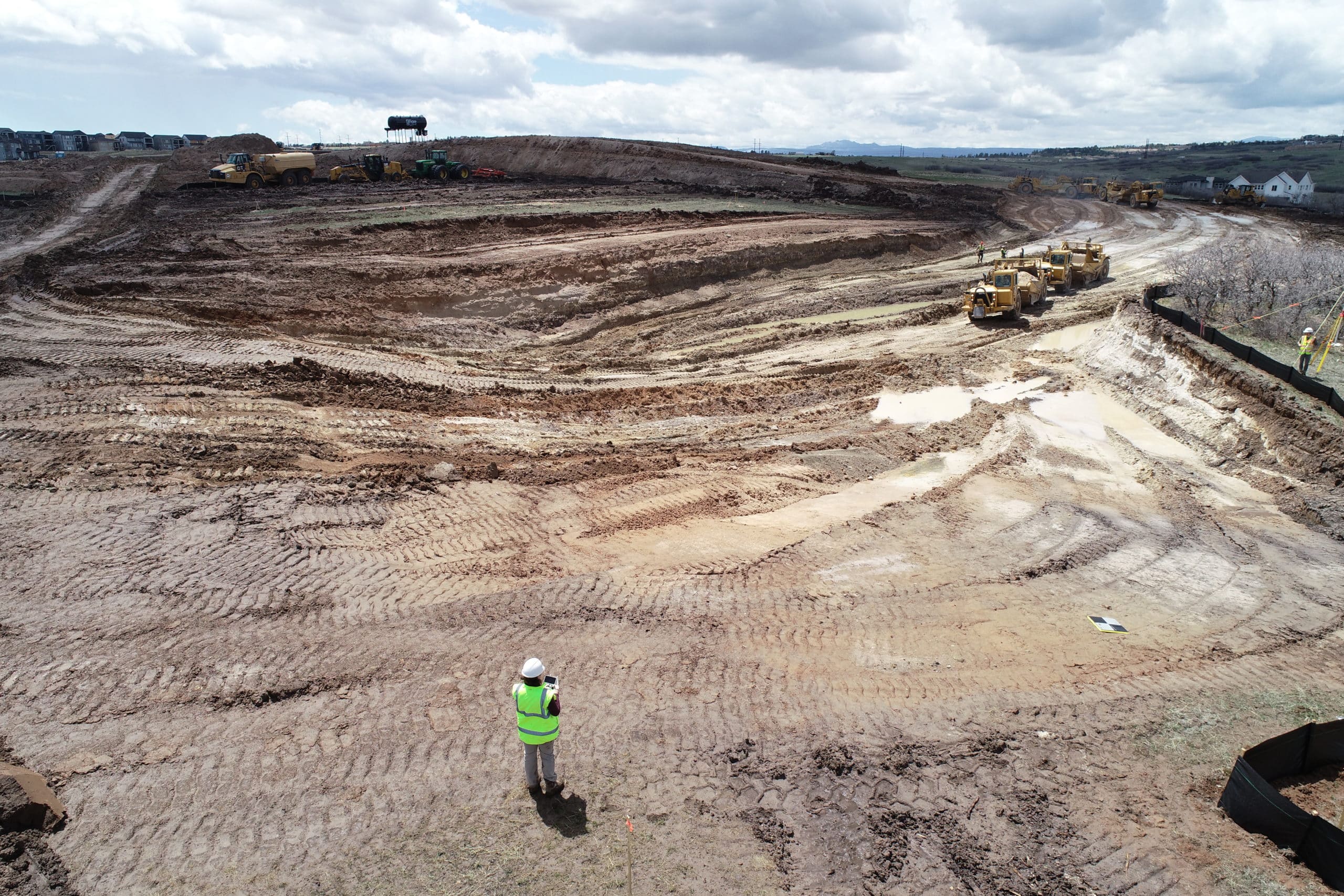This detailed aerial image captures a sprawling construction site, resembling an excavated sand pit or quarry. The vast landscape is marred with deep tire tracks and dotted with puddles of water primarily on the right side. Dominated by tan and brown hues, the soil contrasts sharply with the lush green rolling hills in the background, where a clear blue sky with scattered clouds provides a picturesque backdrop.

In the foreground, a person wearing a neon yellow construction vest with gray stripes and a white hard hat stands, holding something indistinguishable in their hands. Their attire, including jeans and boots, suggests they are a foreman or person in charge, overseeing the site. Beside this individual to the right, a black fence line adds to the structure of the scene, while to the left, rocky outcrops punctuate the vast dirt expanse.

Several heavy yellow construction vehicles populate the area. On the far right, four trucks—some resembling bulldozers or tankers, likely used for soil wetting—drive into the scene, headed towards the solitary worker. Additional yellow and green trucks are parked in the distance on the left. In the backdrop, there are multiple homes, including a notable white house on the right-hand side near the grassy area, hinting at a nearby residential development possibly linked to the ongoing construction project.